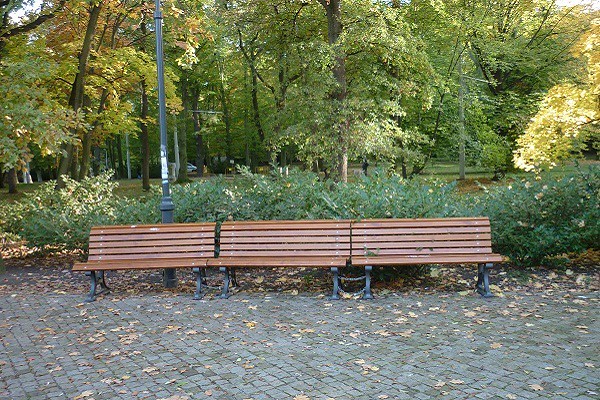The image captures a serene outdoor scene, likely in a city park during early fall. The foreground features a sidewalk area made up of square, stone pavers. Scattered dead brown leaves are evident on the walkway, suggesting the onset of autumn. In a horizontal line along the pavers, three wooden slat benches with metal, cast-iron legs are seen, providing a place of rest. Behind the benches, a neatly trimmed row of green shrubs adds a touch of nature before leading into a background filled with lush, large trees, some slightly turning yellow. A metal pole, likely with a light atop, stands behind the leftmost bench. Subtle details, such as a faintly visible vehicle in the upper left corner and short grass beneath the trees, enrich the scene, making it a picturesque park setting on a crisp, early fall day.